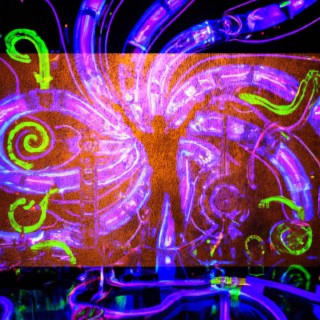The image is a highly vibrant and colorful artwork resembling a neon light poster. The composition is square with thick black borders on the top and bottom, framing a central rectangular space imbued with a bronze, copper-like tone. In the middle of this space is the silhouette of a person, seemingly standing with both arms raised in a celebratory V formation. This figure appears more like a shadow and provides a focal point in the center of the artwork.

Surrounding this silhouette are ten wavy purple lines radiating outward in an "up and to the right" pattern, resembling sound waves. Complementing these are smaller, bright neon green swirls that create a dynamic energy around the central figure. These green lines also appear on the top and bottom within the darker sections and move vertically across the image, adding to the glowing, electricity-like effect.

The top and bottom black borders are punctuated by these vivid color transitions, where purple and blue lines extend from the central red-toned background outward. At the upper part of the image, one prominent green neon line acts almost like an arrow descending into the central space. The bottom left corner features small vertical green streaks against a black background, further adding to the intricate play of light and color.

Together, these elements create a dazzling and energetic scene, with the central figure's silhouette highlighted by swirling, vibrant colors, giving the impression of an electrifying celebration captured in a bright, neon glow.